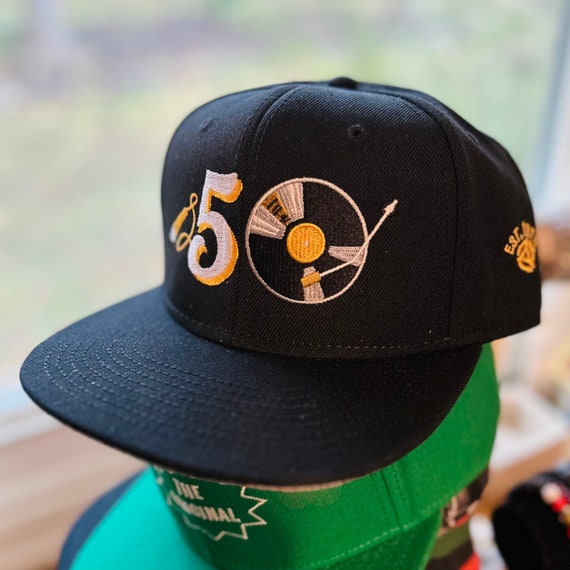The photograph depicts a close-up of two ball caps stacked one on top of the other, taken indoors with natural lighting streaming from a blurred window in the background, suggesting green foliage outside. The image is square, measuring approximately 4 inches by 4 inches. The light brown wood sill of the window is visible at the base. 

The bottom cap is green with the bill facing towards the lower left, partially out of frame. Its front bears the white text "The Original," though some letters are indistinct. On top of it, the black cap faces the same direction. This cap features a prominent white number 5 with a gold outline, giving it a three-dimensional appearance. To the right of the number, an LP record image with a stylus arm is visible, representing the "0" in "50." Gold stitching on the right side spells out "EST," blurring out towards the end. The black cap also has an orange logo on its back side. The background remains out of focus, emphasizing the details of the caps.